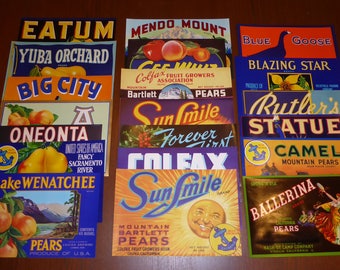This photograph depicts a rich tapestry of vintage produce labels, meticulously arranged on a wooden surface, perhaps a table. The labels are laid out in three overlapping columns, showcasing their vibrant colors and bold typography. At the top left corner, a label reads "Edom" in bright yellow, followed by "Mendo Mount" in red, and "Blue Goose" featuring a small blue goose illustration. Below these, "Yuba Orchard" displays little oranges, though some labels like the possibly "Gee Whiz" one are partially obscured. "Blazing Star" stands out in yellow with an image of a flower, and "Big City" features blue letters against an orange background. Further notable labels include "Colfas, Fruit Growers and Associates, Bartlett Pears," "Oneata," "Sunsmile," and "Statue." This collection, possibly around 20 labels, all shares a vintage charm, reminiscent of the old-style advertisements that adorned walls and bars, primarily highlighting various pear and other fruit producers.